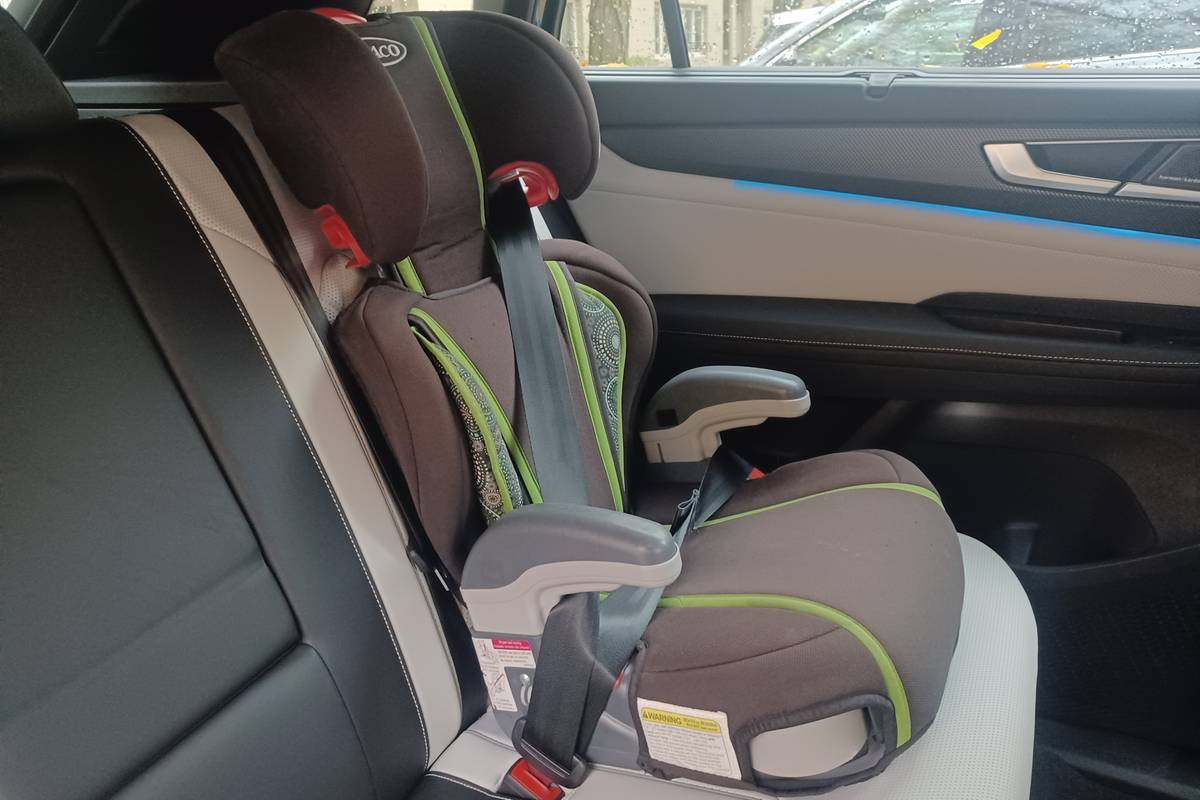The image displays the interior of an SUV, focusing on a child's car seat installed in the rear. The SUV's interior features a mix of black and white leather upholstery, with the back seats showcasing distinctive black and gray paneling on the doors. The child's car seat, which is brown with green trim along the back and front cushions, is securely fastened with the car's seat belt and equipped with red clips near the headrest. The seat is designed for a toddler, as indicated by its size and features. The child seat rests on a white leather seat, and there are visible stickers and a label on the headrest area. The photograph also captures a glimpse of the outside through the car's windows, revealing raindrops and a neighboring parked vehicle.